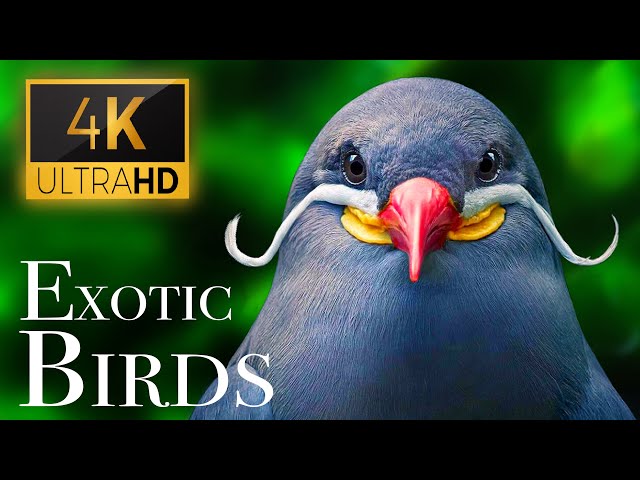An elegant bird, characterized by its distinctive curled moustache-like feathers, gazes out from the image. Its striking yellow mouth appears to be smiling, complementing its vivid red beak. The bird's plumage is a beautiful shade of blue, accentuated by its rounded head and two expressive black eyes. 

Behind the bird, lush green plants form a blurred backdrop, enhancing the bird's prominence in the foreground. 

In the upper left corner, a small square label reads "4K Ultra HD" in yellow and black. Directly below, a white text caption declares, "EXOTIC BIRDS," emphasizing the rarity and beauty of this creature. Both the top and bottom of the photo are framed with black borders, adding a polished finish to the image. 

This detailed caption encapsulates the visual splendor and distinct characteristics of the bird, making it an engaging and informative description.